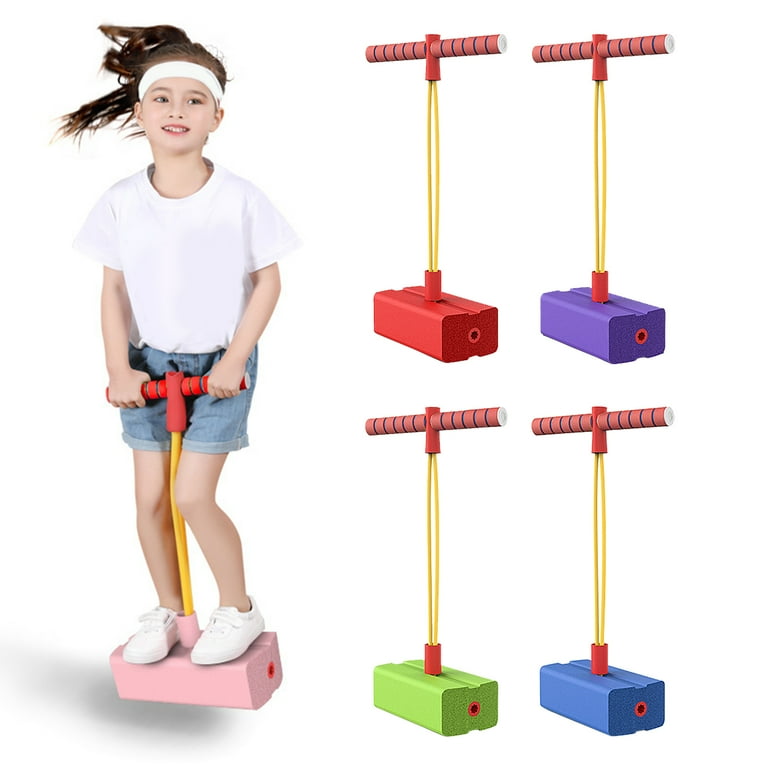In this photograph, set against a white background, a young girl, about nine or ten years old, is captured mid-jump on a vibrant pogo-stick-like toy. The toy features a distinctive design with a long yellow metal bar connecting a brick-shaped footrest and red handlebars. The girl, who has brown hair tied in a ponytail flying behind her, wears a white headband, a white t-shirt, blue denim shorts, and white tennis shoes. Her feet are firmly placed on the pink base of the toy, which seems to be made of a soft foam or rubber material. Surrounding her are four additional identical toys, each differentiated by the color of their footrests: red, purple, green, and blue, all with gold shafts and red handles. The image effectively showcases the toy's colorful variations and playful use, emphasizing its appeal to children.